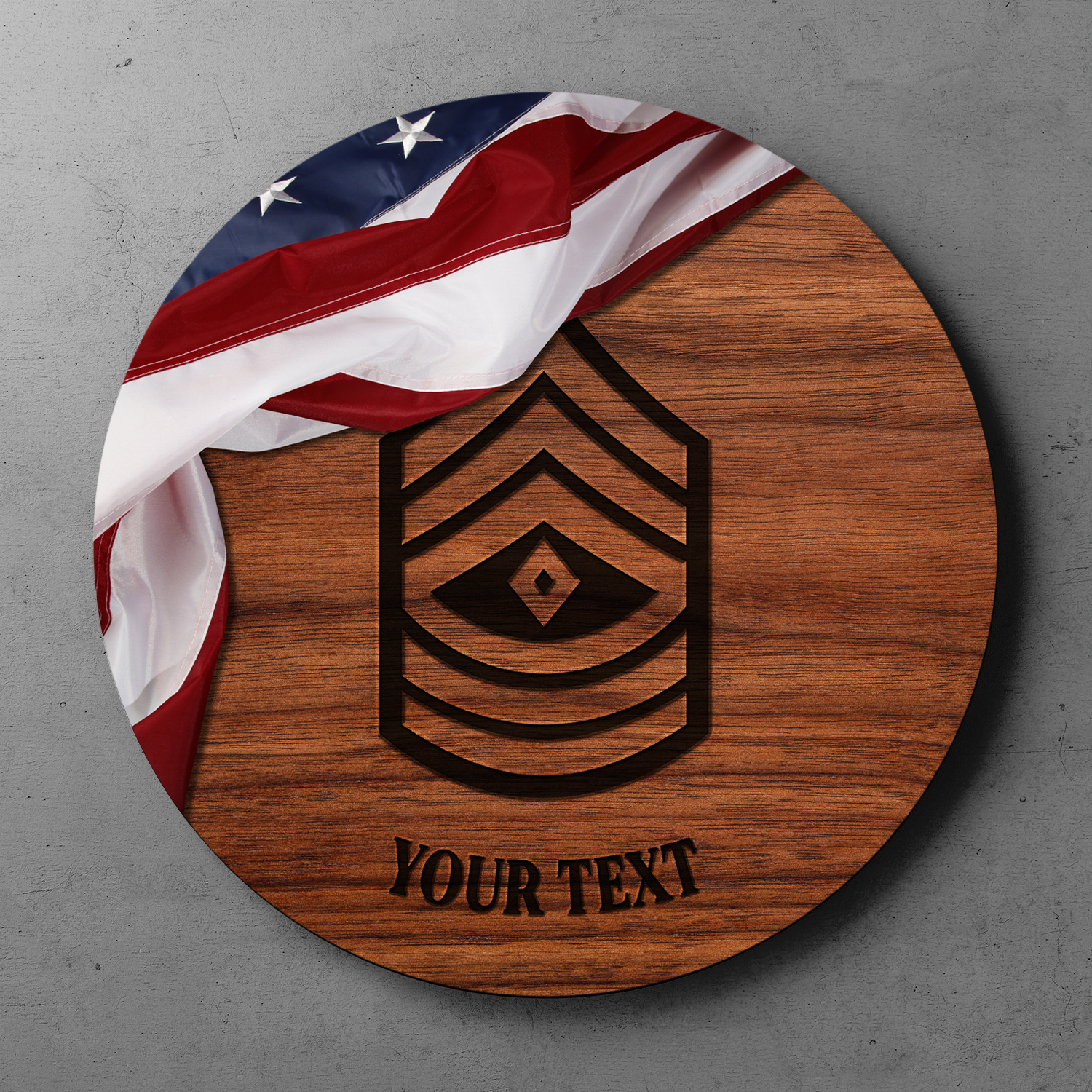The image features a round wooden cutting board adorned with a prominent black logo in the center, reminiscent of a military patch with arrows pointing upward and intricate lines. Below this, in bold black capitalized letters, are the words "YOUR TEXT," indicating that the cutting board can be personalized with custom engraving. Draped over the top left portion of the board is a fabric resembling the American flag, with red, white, and blue stripes and white stars, symbolizing a patriotic or veteran theme. The cutting board is half-covered by this flag-like cloth, revealing its smooth wooden surface. The background of the image is gray, likely a stone or cement surface, with visible shadowing around the product, enhancing its intricate details.